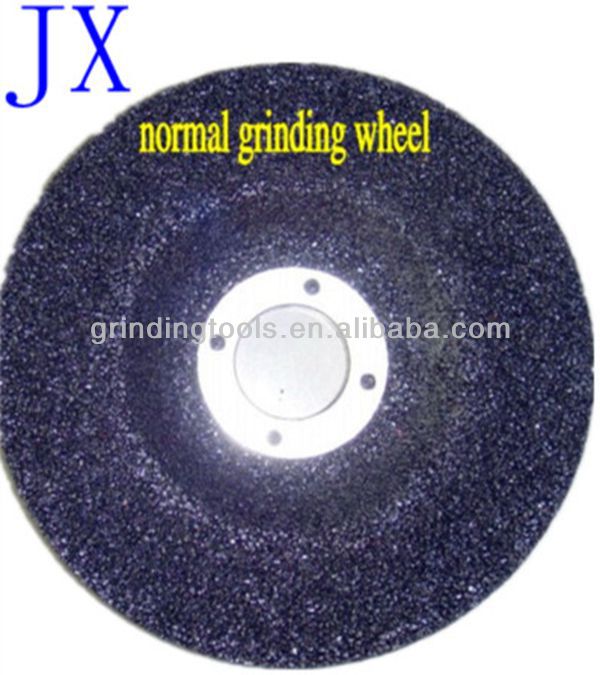This image features a centered, black, round grinding wheel set against a clear white background. The grinding wheel, typically used in construction or automotive industries for cutting, has a visibly coarse texture suited for its purpose. The disc includes a shiny metal mounting plate at its core, with a hole and four round divots for attachment to a grinder. In yellow text at the top of the wheel, it reads "normal grinding wheel." The top left corner of the image shows "JX" in blue font, indicating the manufacturer. Additionally, the center of the image displays the website address, grindingtools.en.alibaba.com, in gray text. This photograph appears to be designed for a sales platform, providing potential customers with a close view of the product's features.